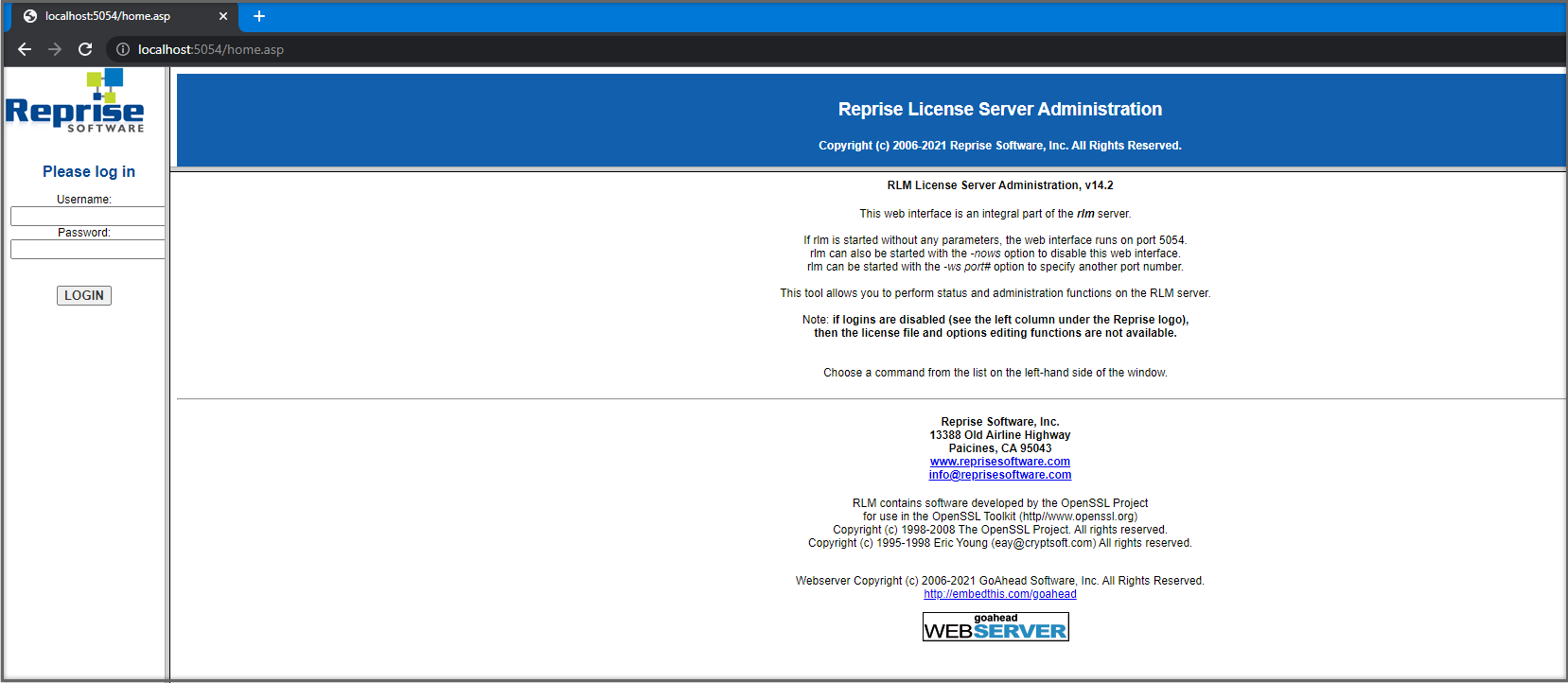**Caption:**

Screenshot of a browser displaying a web interface for Reprice Software's License Server Administration. The browser features a black background header and tab, with the tab labeled "localhost 5054." The address bar also reads "localhost 5054," accompanied by navigation buttons to its left.

The webpage is divided into two main sections:

- **Left Sidebar**: Titled "Reprice Software," it includes the Reprice Software logo, composed of multicolored boxes connected by a line. Below the title, a login prompt asks users to "please login," providing text fields for "Username" and "Password," followed by a "Login" button.

- **Right Panel**: The upper portion of this section has a navy blue background, displaying the text "Reprice License Server Administration" and copyright information dated 2006 to 2001. The middle portion features a white background and states "RLM License Server Administration version 14.2." A bolded note informs users that if logins are disabled, they should refer to the left column under the Reprice logo, mentioning that certain functionalities like license file and options editing are unavailable. The bottom section lists Reprice Software's address, website link, and an email link (info@repricesoftware.com), with a tag at the very bottom center that reads "Go Ahead Web Server."